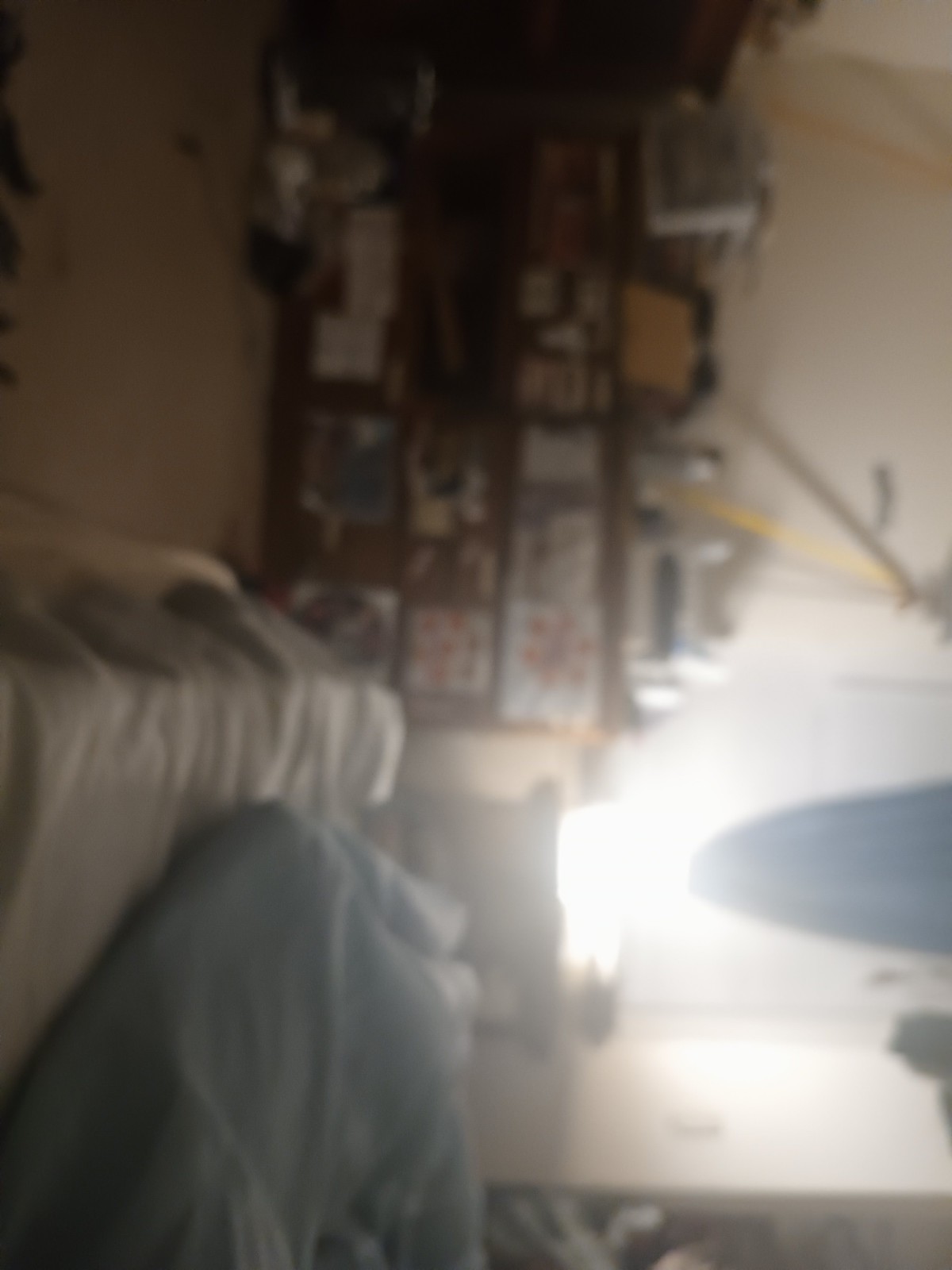The image is a blurry, sideways photograph of a bedroom, rotated 90 degrees from its intended orientation. To view it accurately, you should tilt your head 90 degrees to the right. In the bottom right corner lies a bed covered with a scrunched-up blue duvet and a fitted white sheet. The bed frame is not visible. To the left of the bed, a tan-colored carpet covers the floor. Along the left side of the image (which becomes the top when correctly oriented), there's a series of four shelves filled with indistinct items and a cluttered desktop area. The back of the room features a light source from an electric lamp. A white sheet curtain and a blue drape partially cover the window, allowing a large amount of light to spill into the room. There are multiple stickers or drawings on a cabinet, and a yellow pole is visible near the window. A small table sits beneath the window, contributing to the room’s overall cluttered atmosphere, which resembles that of a teenager’s or child's space.